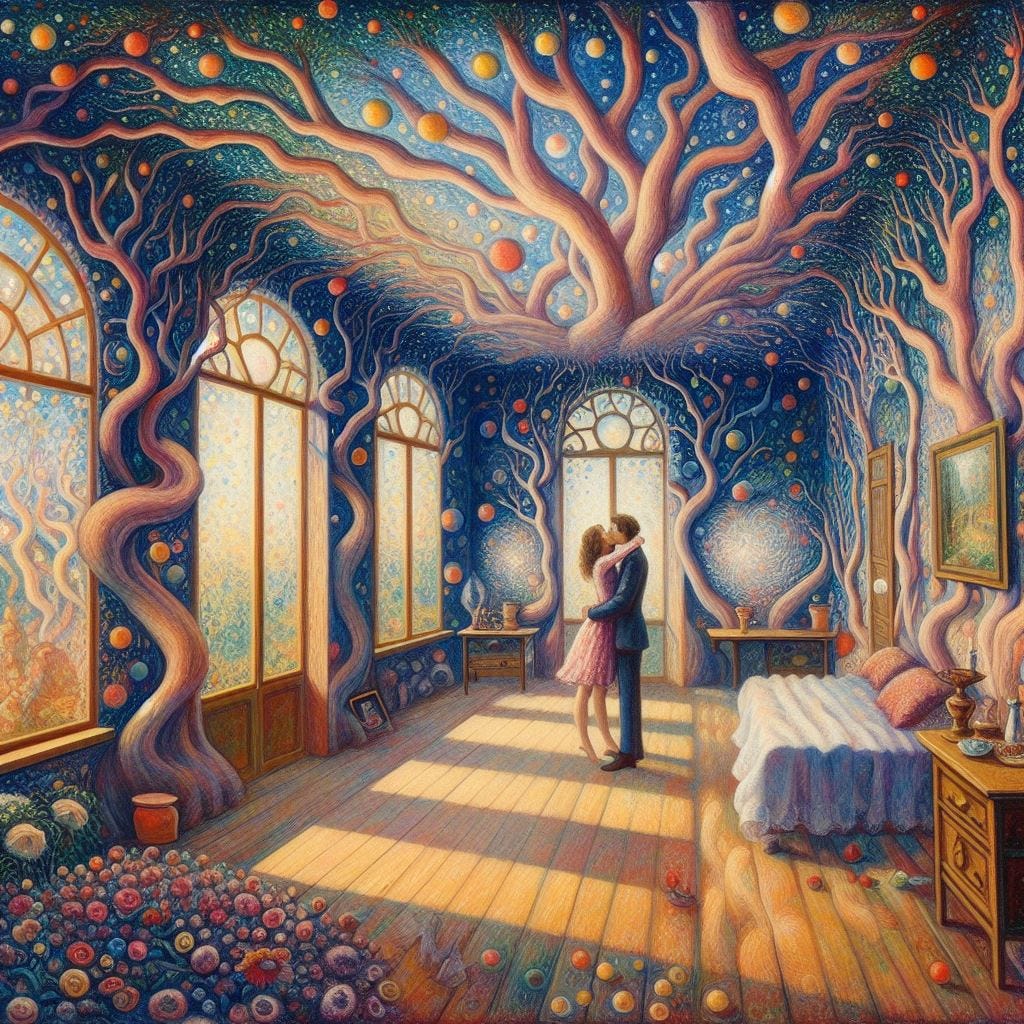This vividly imaginative digital artwork captures an intimate moment between a man and a woman in an enigmatic bedroom. The couple, rendered with meticulous detail, are depicted embracing and kissing, with the woman in a delicate pink dress and the man in a crisp blue suit. The room, adorned with wooden floorboards and blue walls, features several arched windows trimmed with gold, adding a regal touch. Tree trunks and roots emerge from the floor, climbing up and intertwining around the walls and ceiling, creating a surreal and fantastical atmosphere. The ceiling itself is a visual marvel, adorned with swirling branches and roots, interspersed with small, vibrant spheres in shades of orange, yellow, and red, which suggest the concept of space or celestial bodies. The floorscape adds to the whimsical setting with colorful flowers blooming from the left side and these mysterious spheres scattered around, with some resembling small, blooming plants. A small bed with a gold-framed picture above it and a nightstand complete the right side of the room, adding to the homey yet otherworldly ambiance of this striking and detailed digital painting.